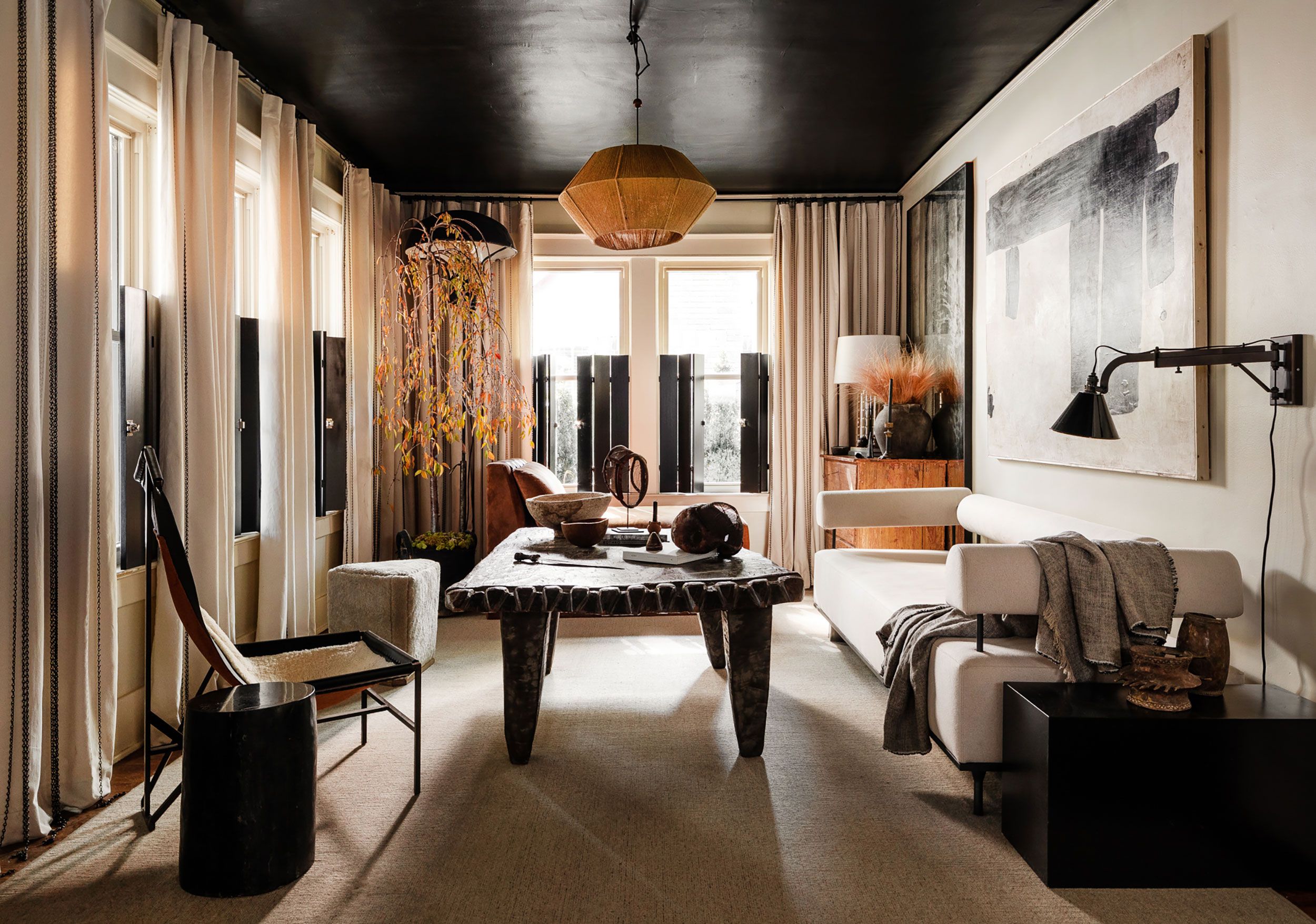This full-color indoor photograph, using natural daylight, captures a modern, sophisticated living room. The image's square format reveals a bright, airy space with large windows adorning the top and left sides, letting in streams of sunlight. The windows are partially covered with elegant wooden shutters on the lower halves and beige curtains framing each side. The ceiling above is a rich, dark brown, from which a stylish overhead light hangs, enhancing the room's upscale vibe. 

In the back of the room stands a tall lamp with a lush green plant in front of it, adding a touch of nature to the modern décor. Central to the composition is a striking table, seemingly crafted from stone with a rock-like texture, adorned with various bowls, a dagger-like knife, and other decorative objects. This table sits on a beige carpet layered over a wooden floor, creating a warm and inviting foundation for the space.

Adjacent to the table is a sleek, white couch with rectangular cushions and cylindrical backrests that appear to float due to thin, cylindrical supports—a testament to the room's modern design. A large black and white abstract painting prominently features on the far-right wall, serving as an eye-catching focal point. Additionally, small desk and standing lamps scattered throughout the room, along with a wooden table and various chairs, round out the furnishings, highlighting the room's blend of contemporary style and cozy ambiance.